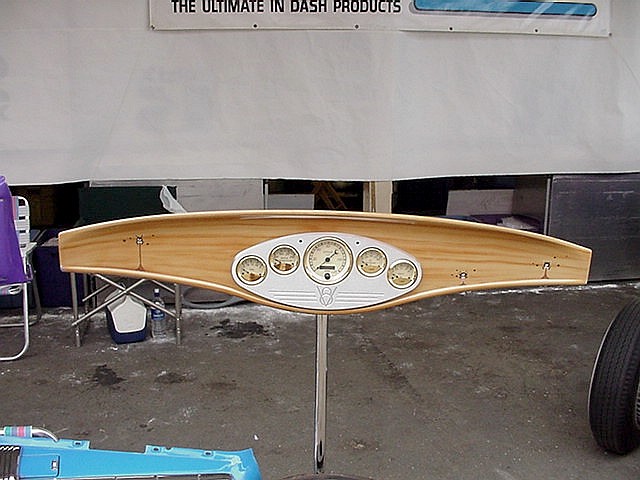This rectangular photograph showcases an outdoor or possibly lit garage setting with a distinctly dim ambiance. The concrete floor, notably dirty with possible oil stains on the left side, forms the foreground. Centrally positioned is a removed dashboard, likely from a watercraft given its design, rather than from a car. This dashboard is horizontally elongated and slightly oblong in shape, crafted from light wood reminiscent of a pine color.

Embedded within the wooden dashboard is an oval-shaped, white metal panel featuring an array of gauges. There are four smaller circular gauges, positioned two on the left and two on the right, and a larger central gauge, likely a speedometer. Beneath this prominent speedometer is an engraving of the letter 'V' flanked by two small circles.

To the left side of the image, there is a partially visible chair, a classic outdoor aluminum foldable type with a white fabric seat and back, and metal aluminum legs and frame. On the right, an Igloo cooler appears in profile, white on the top with a darker color underneath. At the lower left corner of the image, there lies a horizontally positioned, blue metallic piece of equipment, which is otherwise indistinct.